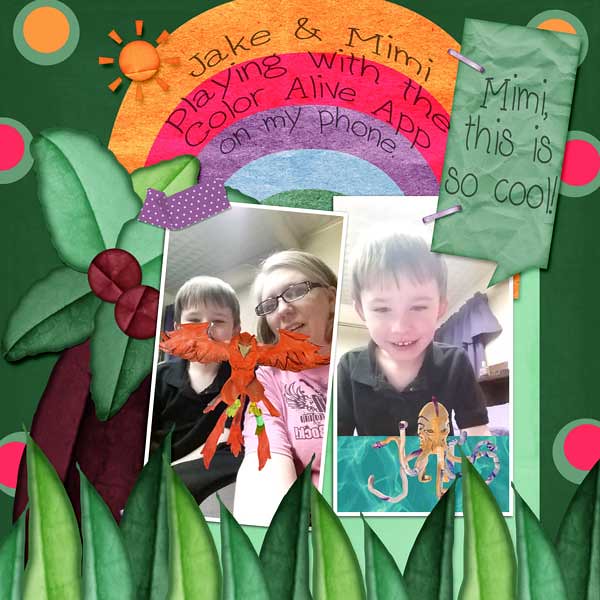A vibrant children's artwork is set against a green background, featuring a colorful rainbow with segments in orange, pink, purple, and light blue. An orange sun beams brightly above the rainbow, and below it, green grass sprouts in the foreground. In the middle of the rainbow, the words "Jake and Mimi playing with the Color Alive app on my phone" are inscribed. Two photographs are superimposed over the rainbow: on the left, an image of a woman and a child, though the child's face is partly obscured by a large, vivid red bird seeming to attack; on the right, likely the same boy looks downward, with an octopus-like creature beneath him and a room with visible curtains and window sills in the background. Additionally, a sticker exclaims, "Mimi, this is so cool!" Bright colors and little red dots enhance the lively scene, suggesting this might be a school project or a fun creation made to show off something special accomplished with the app. The presence of small plants and a palm tree in the backdrop add to the playful and imaginative feel of the artwork.